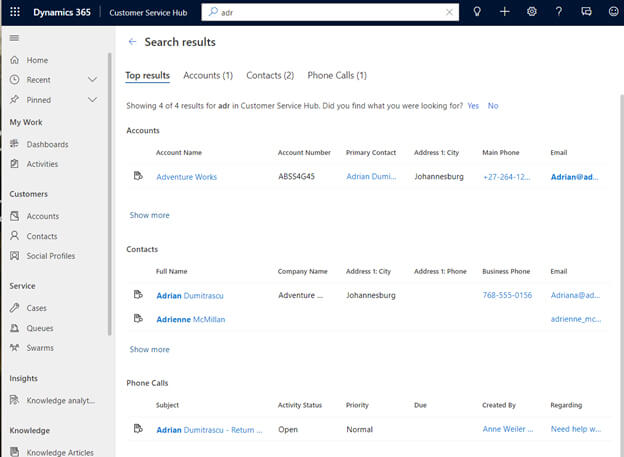Screenshot of a Dynamics 365 Web Page

This detailed screenshot portrays a Dynamics 365 web page within the Customer Service Hub. The layout features a wide gray rectangular sidebar spanning vertically along the left side of the page, while a thinner gray line borders the right side. At the top, a sleek black banner stretches across the page, prominently displaying a centrally-located search bar with a contrasting white background.

On the left-hand sidebar, a comprehensive list of navigation options is displayed vertically. These options include: Home, Recent, Pinned, My Work, Dashboards, Activities, Customers, Accounts, Contacts, Social Profiles, Service, Cases, Queues, Swarms, Insights, Knowledge Analytics, and Knowledge Articles.

The search results for "ADR" are prominently shown within the main content area, focusing on the Customer Service Hub. The results feature highlights related to "Adventure Works" and include specific contacts such as Adrian Dumitrassoy and Adrian McMillan. Additionally, the search results display phone calls associated with Adrian Dumitrasco, providing a rich context for the information being accessed.

This detailed composition enables users to navigate efficiently through the Dynamics 365 platform, providing an organized and user-friendly experience centered around customer service management.